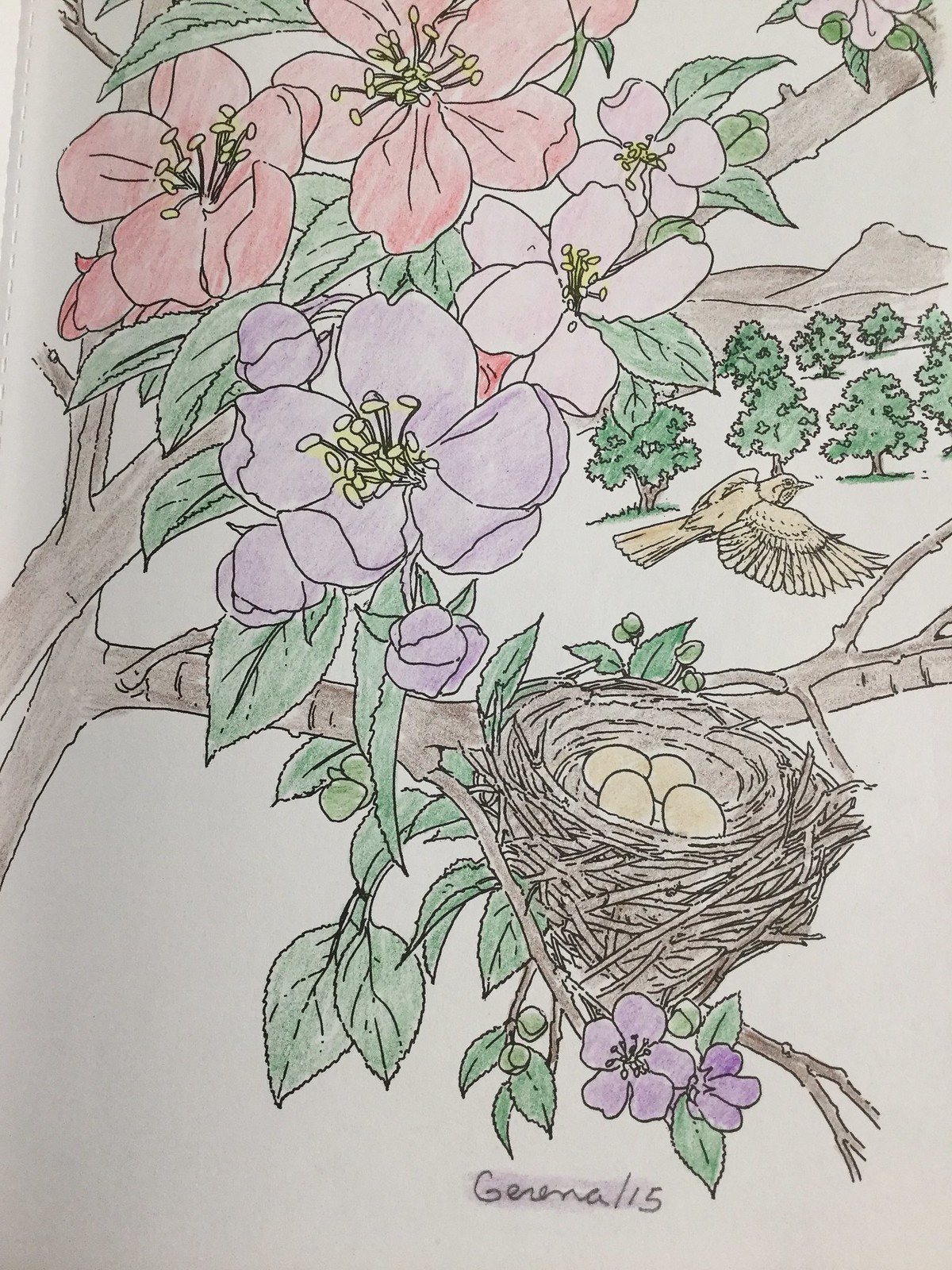This image vividly captures an illustration on a piece of off-white paper, reminiscent of a page from a coloring book, defined by black outlines. At the center of the illustration is a tree branch with two intertwining boughs, shaded in a dark grayish brown hue. Resting on the branch is a bird's nest containing four light yellowish-brown eggs. 

Surrounding the nest are graceful leaves adorned with vibrant purple flowers and occasional fruits, uniformly painted in a green shade. Interspersed among the foliage are two striking red flowers and additional purple ones, totaling approximately five. 

In the backdrop, on the right side, the ground and a mountainscape extend into the distance, both rendered in earthy brown tones. A field of trees enhances the distant horizon. Notably, a bird, colored in the same light hue as the eggs, is seen flying away from the nest, suggesting it may be the mother bird. 

Adding a personalized touch to the artwork is a childlike signature at the bottom right, inscribed as "GERENALIS." The paper's texture and appearance are akin to typical coloring book paper, contributing to the overall impression of a hand-colored, whimsical scene.